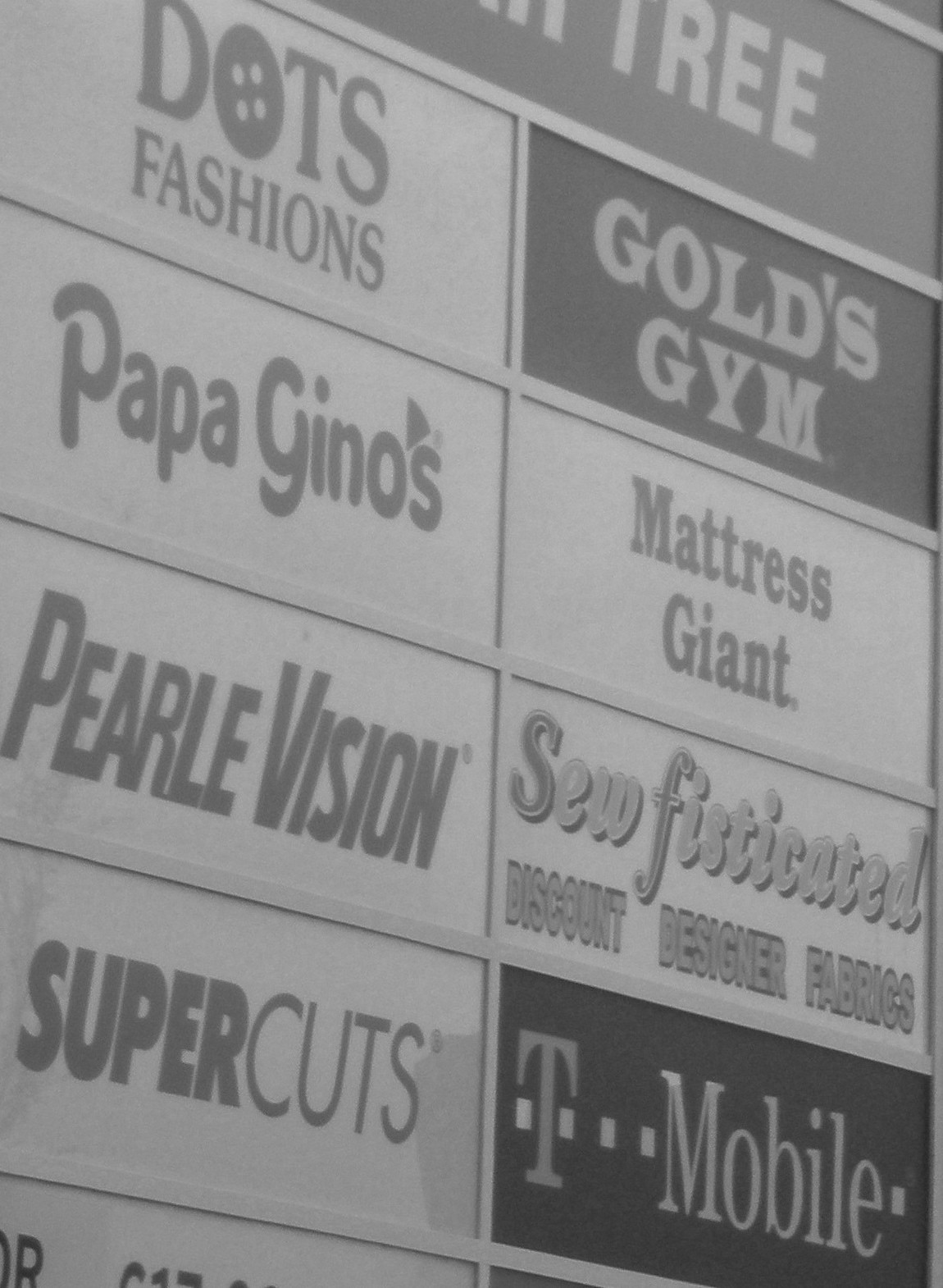This black-and-white, low-resolution photo captures a sign outside a strip mall or shopping plaza, listing various businesses. The sign is dominated by a large, partially visible "Dollar Tree" logo at the top. Below it, the sign is divided into two columns of smaller rectangles.

On the left column:
- **Dots Fashion**, with its distinctive button-shaped "O."
- **Papa Gino's**, identifiable by a small piece of pizza above the "S."
- **Pearl Vision.**
- **Supercuts.**
- An unreadable name obscured at the bottom.

On the right column:
- **Gold's Gym.**
- **Mattress Giant.**
- **Sophisticated Discount Designer Fabrics**, with "Sophisticated" spelled creatively as "S-E-W-F-I-S-T-I-C-A-T-E-D."
- **T-Mobile.**

The image, devoid of people and focused solely on the sign, offers a clear and detailed view of the business names and some iconic logos, albeit in monochrome.